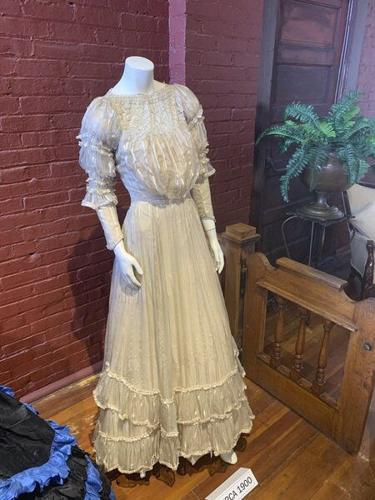This image depicts a detailed display in a museum, featuring a white, off-white, or cream-colored lace dress from the early 1900s, possibly a wedding dress. The long-sleeved dress has a frilly bottom and slightly puffy sleeves that taper off toward the hands. The display, standing on rich hardwood floors, is bordered by a small wooden railing with a lock. A plaque in front of the dress reads "circa 1900." To the left, partially visible, is another dress described as black with blue fringe, which might be a hoop skirt extending to the floor, typical of what women wore in saloons. A green fern in a bronze planter is situated to the upper right of the dress display. The ambiance is marked by the red brick walls of the building, enhancing the historical presentation of the dresses with shades of brown, white, blue, and black.